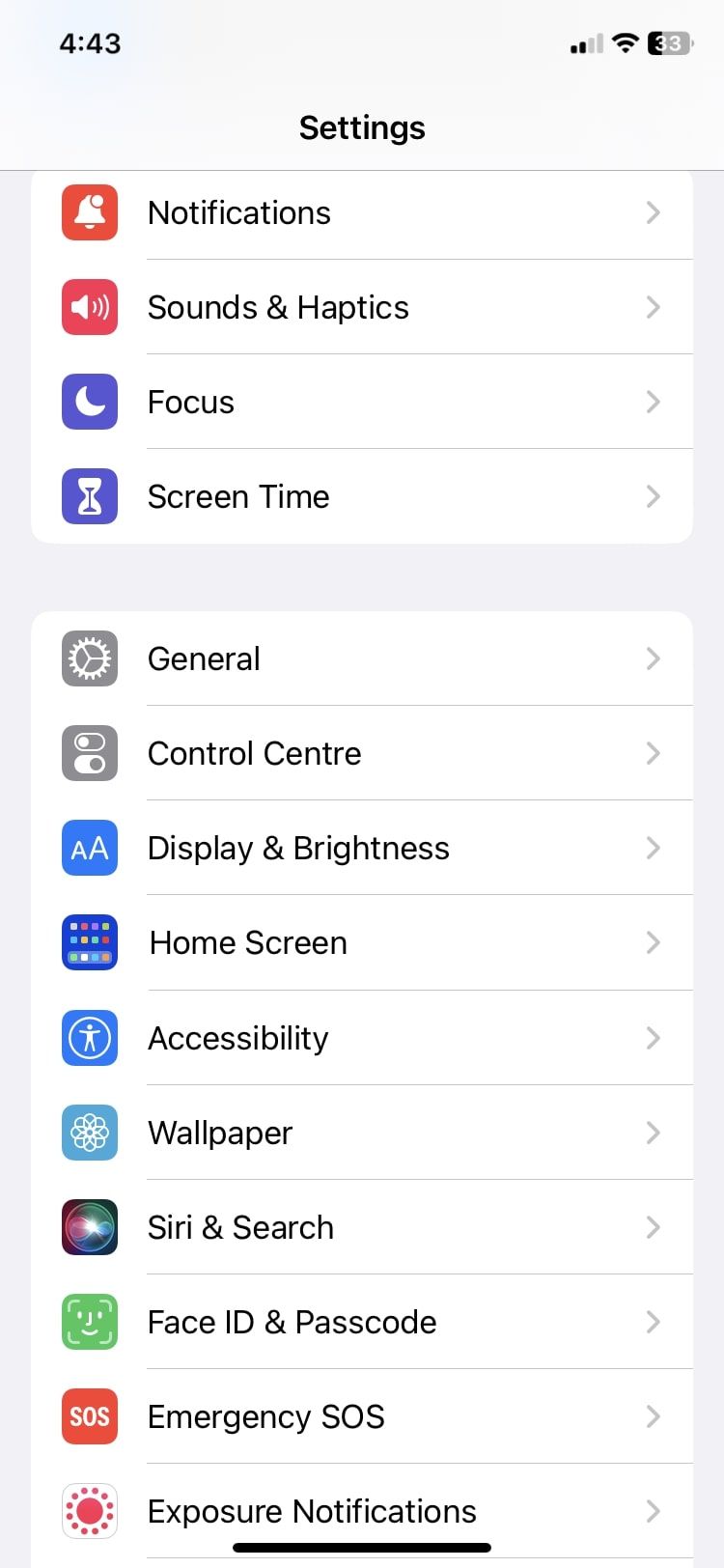This screenshot displays the settings screen of an Apple iPhone, providing a detailed view of various configuration options. Centered at the top of the screen is the title "Settings." Below the title, multiple categories are listed vertically, each housed within white boxes that span the width of the screen.

The first white box contains four options:

1. **Notifications** 
2. **Sounds & Haptics**
3. **Focus**
4. **Screen Time**

To the right of each option, there is a small gray arrow pointing to the right, indicating the ability to expand these categories for additional settings.

Following the initial white box, there is a larger white box encompassing several more options:

1. **General**
2. **Control Center**
3. **Display & Brightness**
4. **Home Screen**
5. **Accessibility**
6. **Wallpaper**
7. **Siri & Search**
8. **Face ID & Passcode**
9. **Emergency SOS**
10. **Exposure Notifications**

Each of these options also features a drop-down arrow to the right, though none are expanded in this view.

At the very top left of the screenshot, the current time is displayed. To its right, a series of icons provide additional information about the phone's status, including the Wi-Fi signal, cellular signal strength, and the battery percentage. 

Overall, the screenshot encapsulates a well-organized array of settings, offering a comprehensive overview of the customization and functional options available on the device.